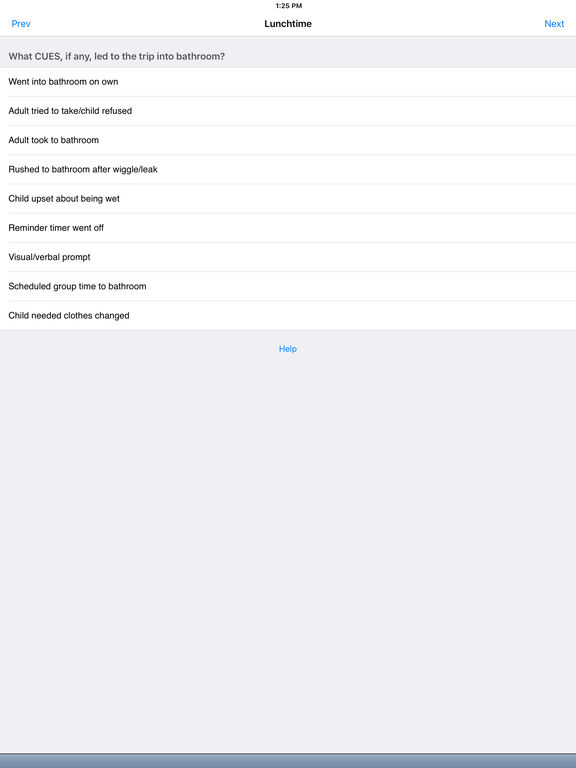This image depicts a detailed record-keeping page designed to monitor and document a child's bathroom visits, particularly focusing on toilet training challenges. The page includes various prompts and headings such as "What cues, if any, led to the trip to the bathroom?" and categories like "Went into bathroom on own," "Adult tried to take, child refused," "Adult took to bathroom," "Rushed to bathroom after wiggle leak," "Child upset about being wet," "Reminder timer went off," "Visual/verbal prompt," "Scheduled group time to bathroom," and "Child needed clothes changed." These entries help caregivers systematically track the child's toileting habits, noting any issues with urinary or bowel incontinence, and identifying cues or interventions that triggered bathroom visits. This structured diary serves as a tool for understanding and addressing the child's potty training progress and challenges.